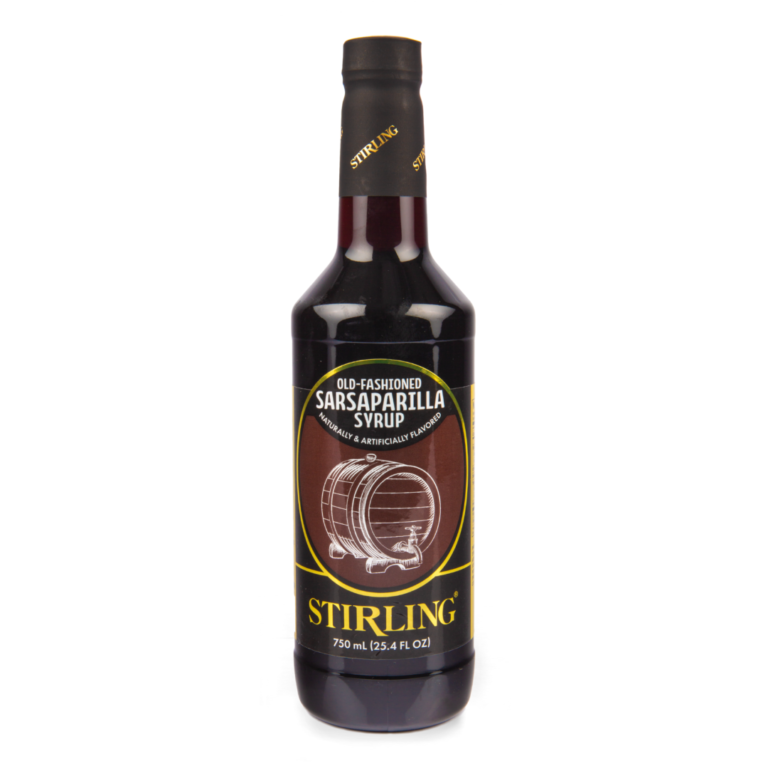The image depicts a dark, almost black, opaque glass bottle of old-fashioned sarsaparilla syrup, branded "Stierling." The bottle's neck is sealed with a dark gray, charcoal-colored wrapper. The label is an oval shape with a gold outline and a black background, featuring the brand name "Stierling" printed diagonally in gold. Central to the design on the label is a large, sideways barrel set against a brown-maroon background. The text on the label reads "Old-Fashioned Sarsaparilla Syrup" followed by "Naturally and Artificially Flavored." The capacity of the bottle is indicated as 750 milliliters (25.4 fluid ounces). The bottle stands alone in front of a white background, and its rich, detailed features suggest a realistic and classic presentation.